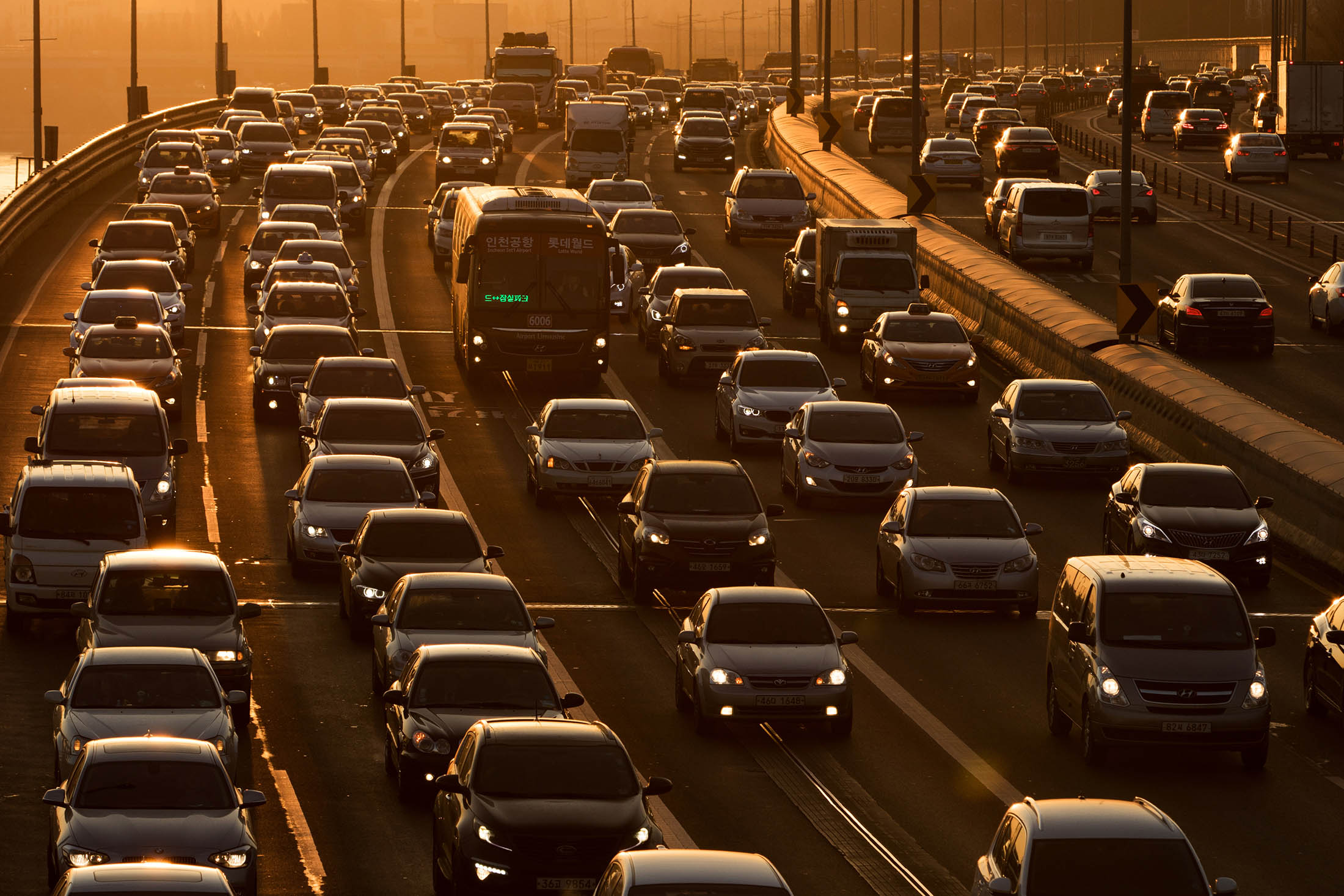The image is a landscape-oriented, color photograph bathed in a golden-yellow hue, suggesting it was taken during either sunset or sunrise. The scene vividly captures a busy freeway, likely in a major city, filled with an immovable traffic jam. The photograph is taken from an elevated vantage point, revealing five lanes on the left, filled with cars, trucks, and buses, all traveling towards the viewer with their headlights on. The presence of vertical struts and a guardrail curving right indicates that this section of the freeway is on a bridge. A concrete central divider with vertical struts separates the oncoming traffic from the lanes moving away, which are partially visible and appear to consist of at least two lanes. The road, dark and monochrome, is flanked by vehicles almost bumper to bumper, adding to the sense of congestion. A thick, smoggy atmosphere adds a layer of haze to the scene, with faint text in an unreadable language on the bus, possibly Korean. The overall composition conveys the immensity of the traffic and gives off a somber yet serene quality due to the golden ambient light.